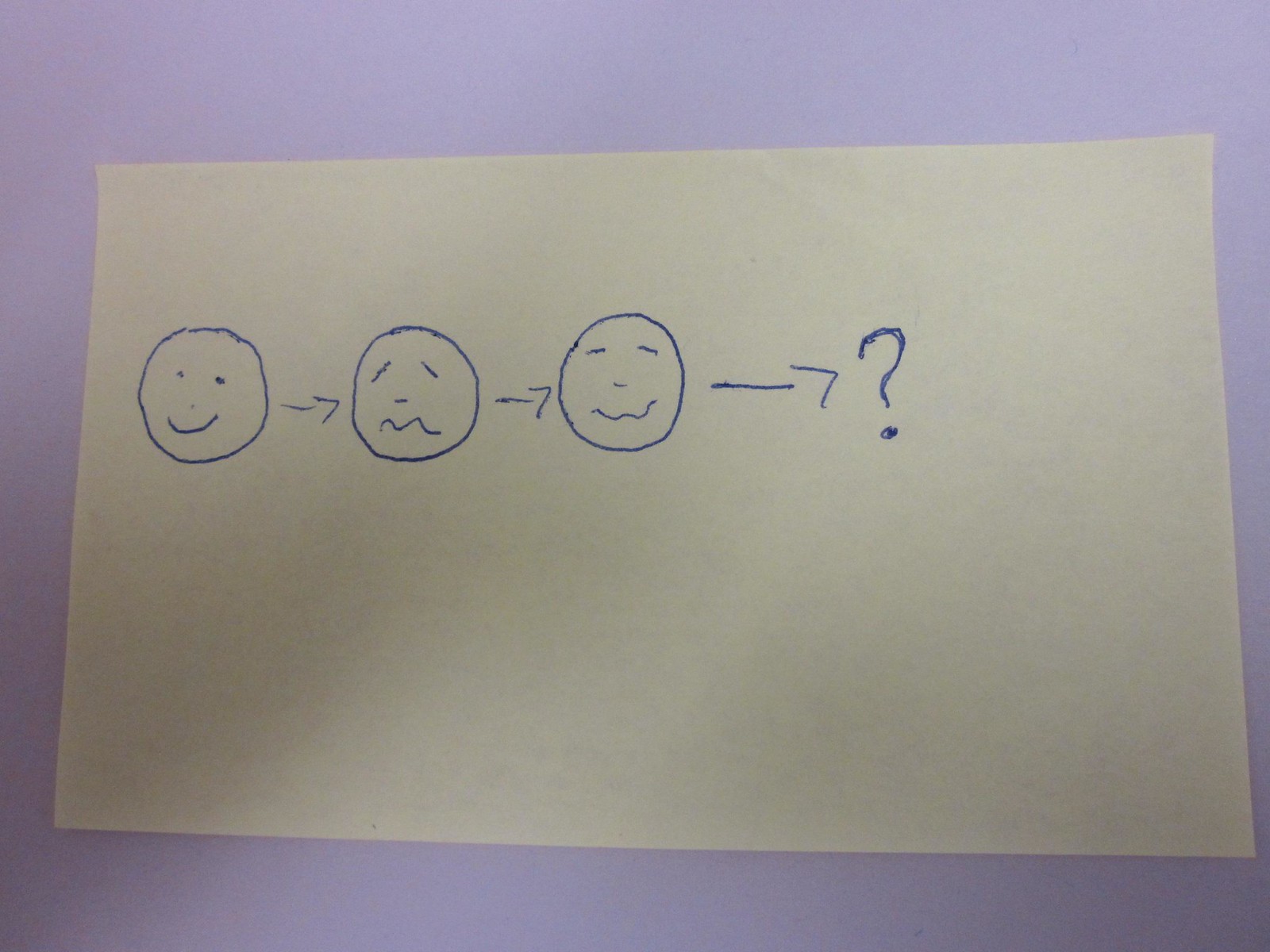The photograph captures a piece of white school paper featuring noticeable grain, set against a light purple lilac-colored background. The paper is oriented in a landscape position. On its left side, there is a series of pen drawings. The first drawing is a crudely rendered smiley face with two dots for eyes, a faint dot for a nose, and a simple curved line for a mouth. An arrow from the smiley face points to a second drawing, a sad face, characterized by diagonally oriented eyes, a straight line for a nose, and a squiggly line for a mouth. This sad face is connected by another arrow to a third face, which has straight lines for eyes, a slightly curved line for a nose, and a wavy, smiling mouth. Finally, an arrow from this face leads to a prominently drawn question mark, outlined multiple times in blue pen, featuring a bold dot at its base. The arrangement casts subtle shadows on the paper, adding depth to the overall composition.